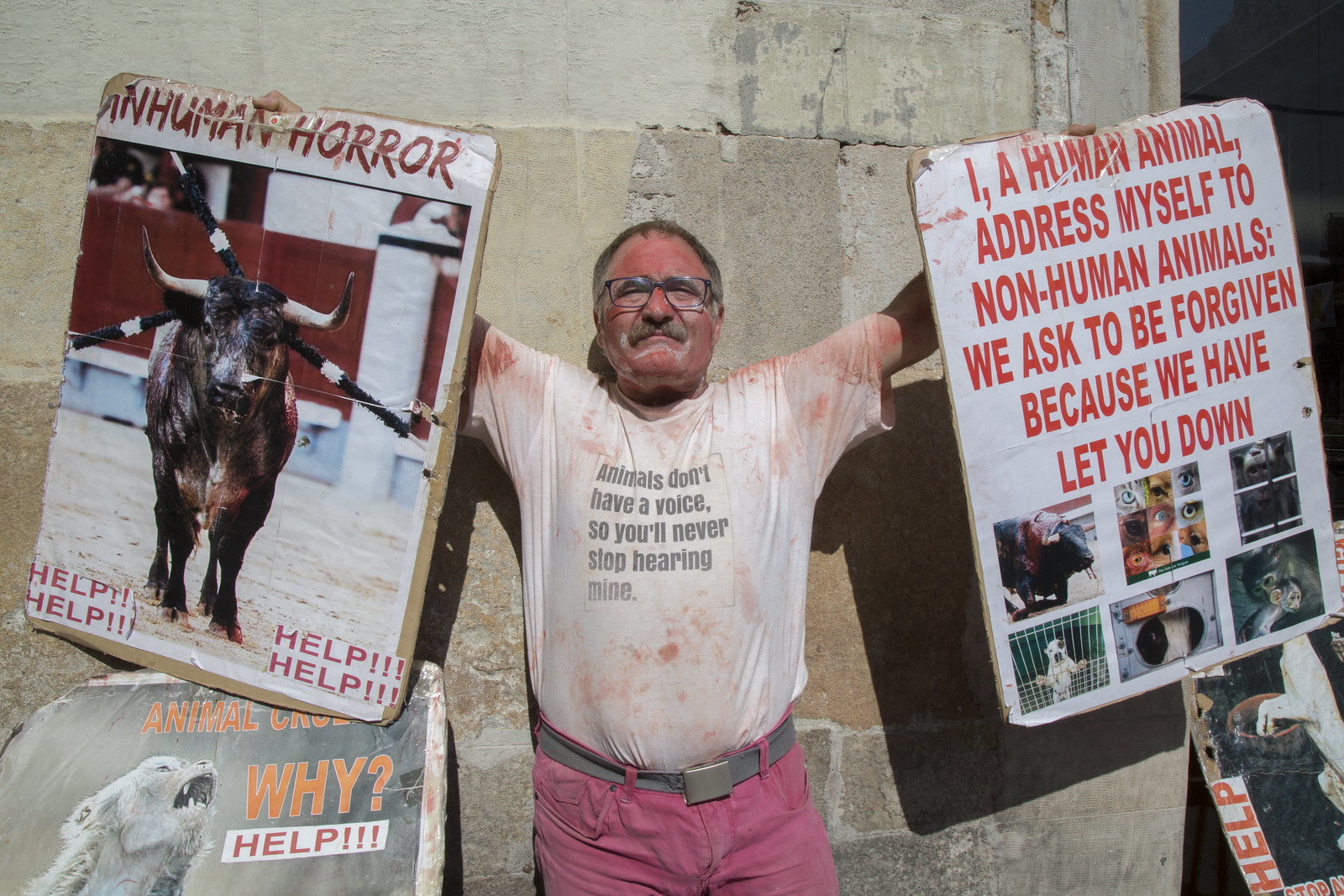The image depicts an older man, possibly in his late 40s, standing outside in front of a cement or stone wall. He has a mustache, glasses, short hair, and is wearing a white shirt heavily stained with what appears to be fake blood. The shirt prominently displays the message, "Animals don't have a voice, so you'll never stop hearing mine." He is dressed in red or pink pants and is holding up two large signs, one in each hand.

The sign in his right hand reads, "Inhuman Horror," with a disturbing image of a bull, potentially related to bullfighting, bull roping, or bull riding. The bottom of the sign repeats the word “Help” four times. The sign in his left hand features the text, "I, a human animal, address myself to non-human animals. We ask to be forgiven because we have let you down." Below this text are six small photographs: one depicts a monkey in a cage, another shows a dog in a cage, and others likely illustrate animals suffering, possibly used for testing or entertainment, though some images are not clearly discernible.

Lying on the ground beside him are additional signs, similar in nature to those he's holding. The scene clearly portrays the man as an animal rights activist, passionately protesting and advocating for animal welfare amidst a backdrop symbolizing confinement or imprisonment.